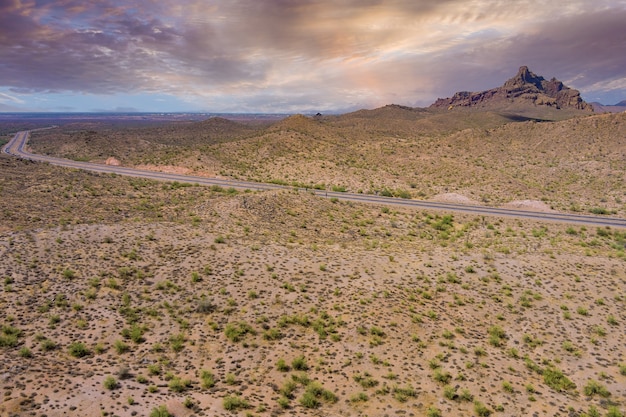The photograph beautifully captures a quintessential desert landscape, reminiscent of the American Southwest. Dominating the scene is a two-lane highway that slices through the barren, sandy terrain, adorned with sporadic tufts of green desert scrub. The road begins at the midsection and travels straight before curving leftwards towards the horizon. To accentuate the austerity of the land, a prominent mesa or rocky bluff stands in the distance on the upper right-hand corner, adding a sense of majesty to the flat expanse. The sky, occupying three-quarters of the upper portion of the image, showcases low-lying clouds through which the sun subtly peeks. These clouds exhibit varying tones – with illuminated sections tinged in yellow-orange, contrasting sharply against the shadowed, darker parts. The undulating, hill-like formations punctuate the otherwise flat desert, creating a sense of depth and texture in this breathtaking desert panorama.